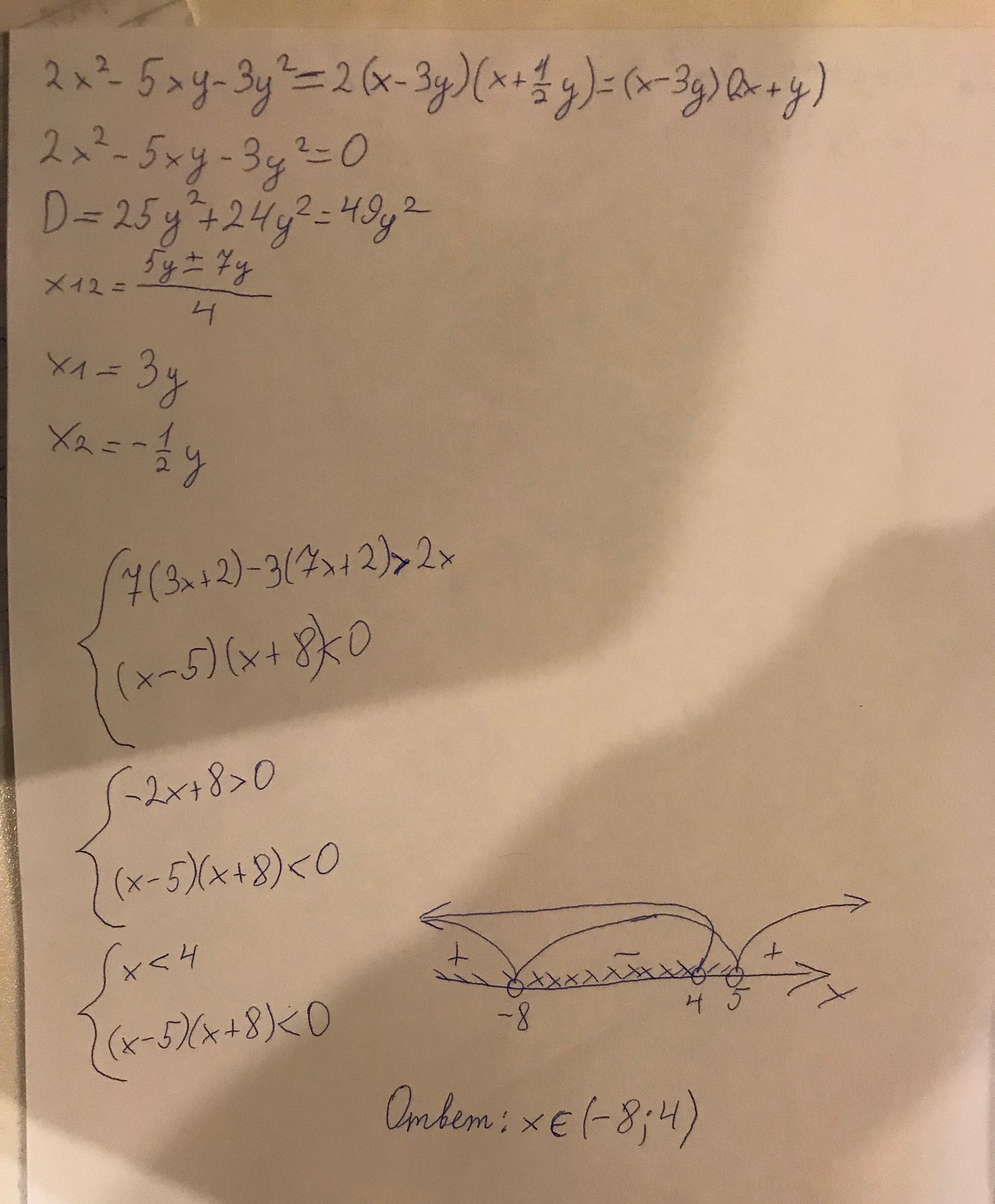This photograph captures a white sheet of paper filled with algebraic equations, all handwritten in blue ink. At the top of the page, there is a quadratic equation that reads: "2x² - 5xy - 3y² = 2(x - 3y)(x + ½y) = (x - 3y)(2x + y)." The equation is meticulously expanded and factored. Below this quadratic equation, several lines of detailed calculations are shown, determining the values of x₁ and x₂ in a methodical step-by-step process spanning six lines. Further down the page, additional algebraic workings are presented, accompanied by a neatly drawn number line. Towards the bottom of the page, there is a complex expression: "OMBEM: times e(-8); 4(...)," which appears to be part of the final solution to the mathematical problem presented. The sheet reflects a thorough exploration and solution of multiple algebraic problems, capturing the precision and effort involved in solving advanced mathematics.